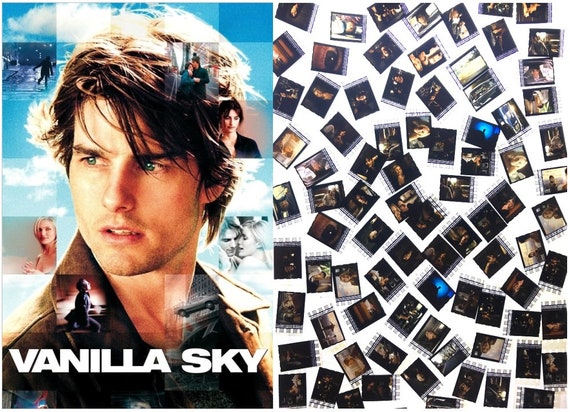The image showcases a visually striking movie poster for "Vanilla Sky," starring Tom Cruise. Dominating the left side, Tom Cruise's portrait captures him with tousled brown hair and a focused look to his left. His face, the central element, is superimposed with various smaller images of women and other scenes from the movie, creating a double-exposure effect. To the right, a cluster of Polaroid-style pictures, showcasing fragments of different scenes and characters, adds a mosaic-like texture. The primary background is a vibrant blue sky dotted with white clouds, emphasizing the movie's ethereal theme. At the bottom, the title "Vanilla Sky" appears in white font, seamlessly blending with the poster’s overall color palette of blues, browns, and whites. The intricate collage of images, combined with the dramatic depiction of Tom Cruise, makes the poster an engaging and intriguing piece of advertising.